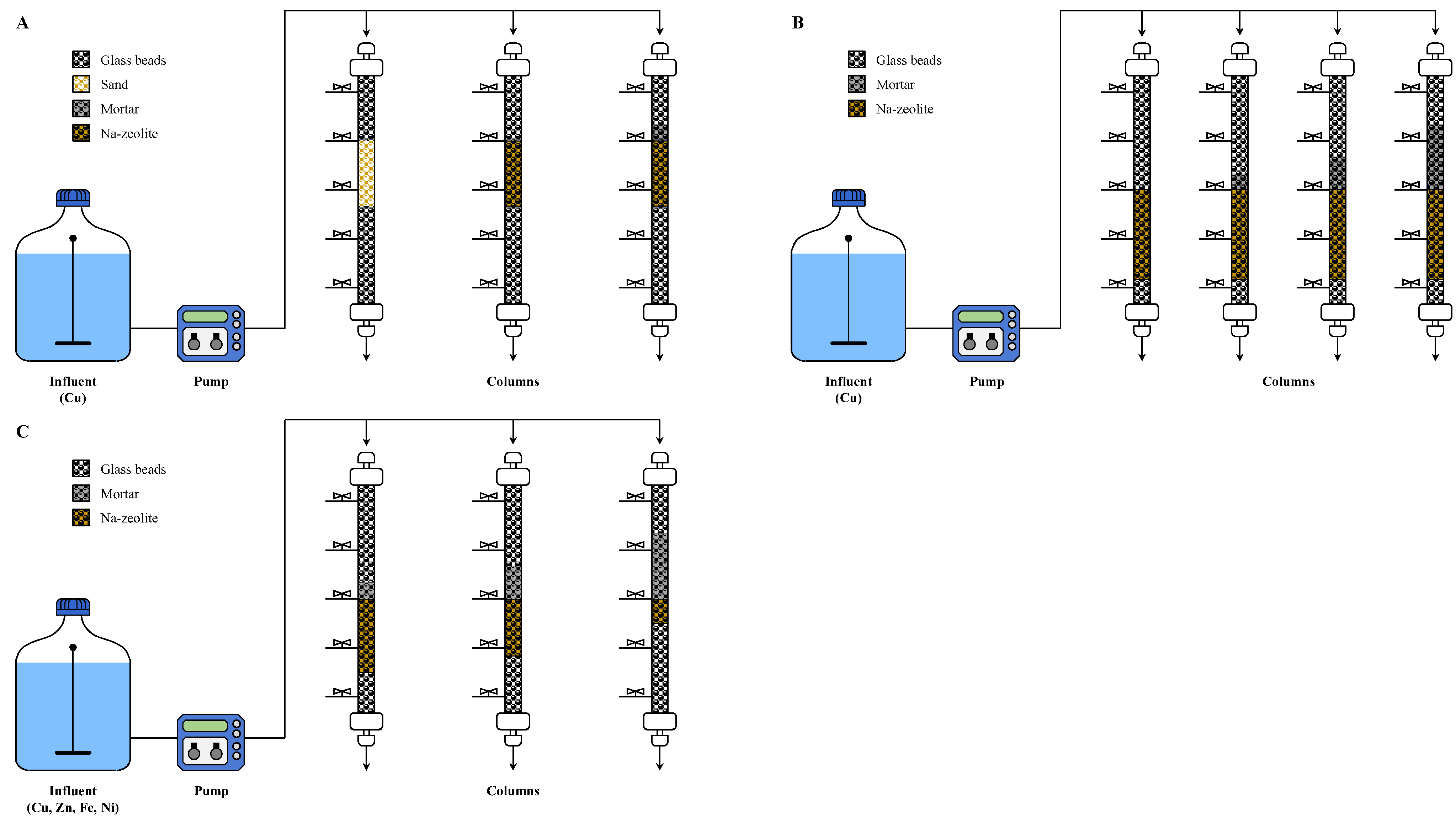This image features a set of three detailed technical schematics labeled A, B, and C, organized with two diagrams on the top row (A and B) and one on the bottom left (C). Each diagram contains a prominent large bottle filled with a blue liquid, labeled "Influent (CU)" with a blue cap. This bottle connects via a line to a small blue box labeled "Pump," which then feeds into multiple columns through a complex piping arrangement. Small arrows indicate the flow direction to three gauges in each diagram.

All three diagrams depict columns containing different materials indicated by specific shading on a black-and-white checkered background. These materials, which are listed in a legend at the top left, include glass beads (gray), sand (yellow), mortar (dark gray), and non-zeolite (dark brown).

In Diagram A, three columns are filled with varying proportions of glass beads, sand, mortar, and non-zeolite. Diagram B features four columns but only with glass beads, mortar, and non-zeolite in differing amounts. Diagram C, similar to A in its basic layout, but unlike B, contains three columns filled with only glass beads, mortar, and non-zeolite.

Each column in the schematics is equipped with white valves at both the top and bottom, highlighting control points for the flow within the system. The emphasis on the shared elements such as the bottle, pump, and columns, along with the differences in material composition, is key to understanding the depicted processes and their variations.